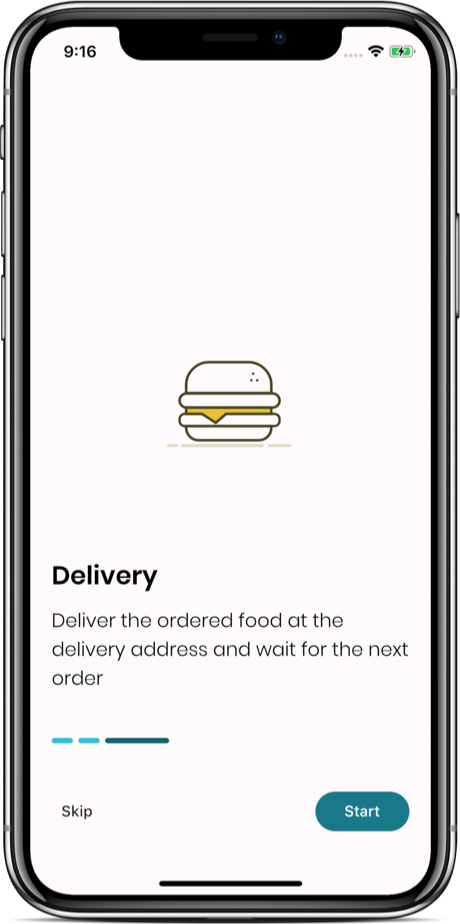The image showcases the front view of a smartphone. The top portion of the screen features a white background. In the top left corner, the time is displayed as "9:16" in black. On the right side, icons for Wi-Fi and battery status are visible. Dominating the upper section of the screen is ample white space, with a central graphic of a stylized hamburger outlined in black. The middle of the hamburger is filled with a yellow element, resembling cheese, nestled between the two buns.

Beneath the graphic, more white space is present, followed by bold black text on the left side that reads "Delivery." Directly below this, a smaller and less bold text provides instructions: "Deliver the ordered food at the delivery address and wait for the next order."

Moving further down, there are three oval-shaped progress bars: two short turquoise bars and one longer bar in a dark greenish-blue hue. Following a small section of white space, the word "Skip" appears in black text. Positioned on the far right side is a bluish-green button with the word "Start" prominently displayed in white text.